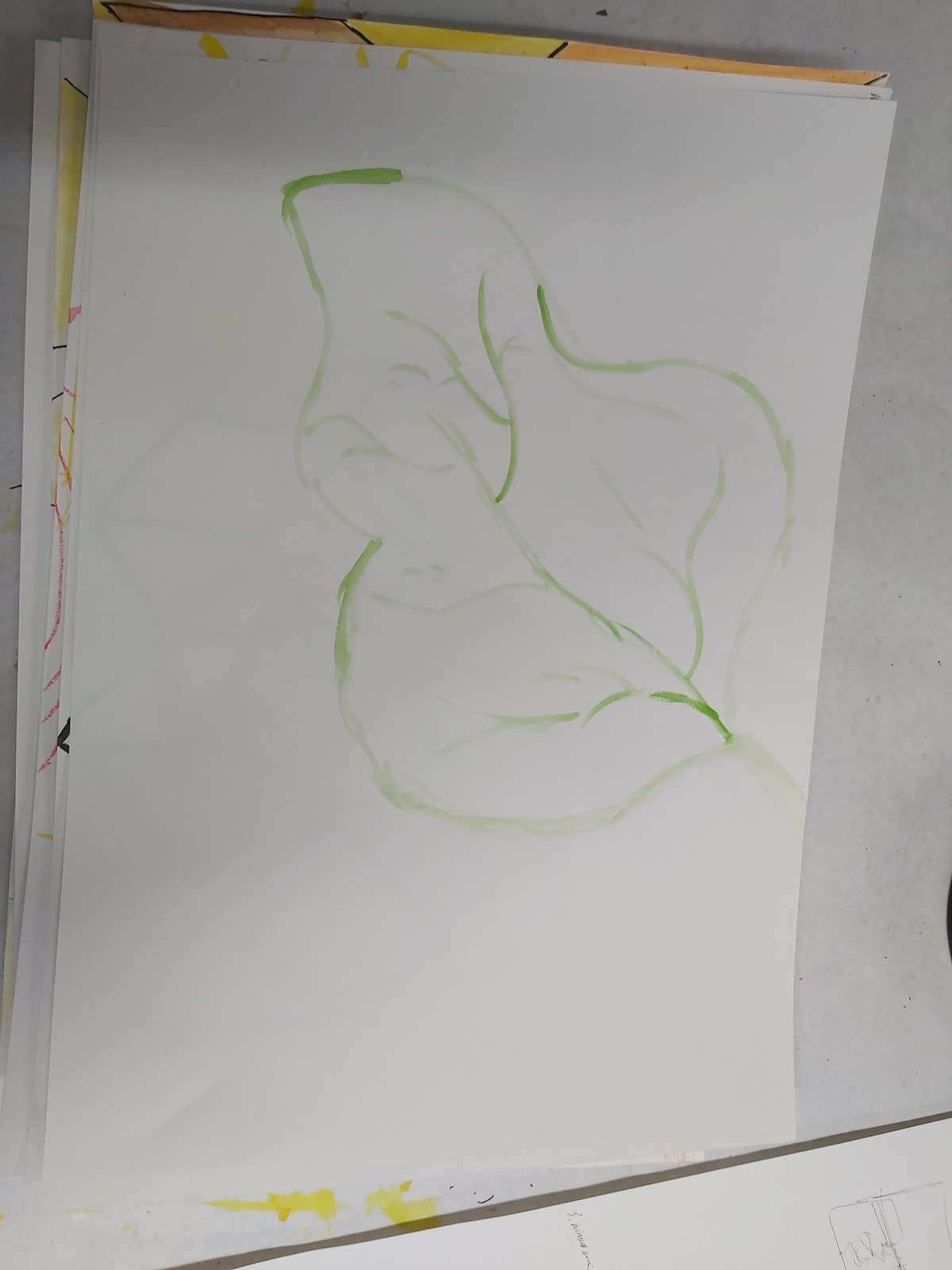The photograph captures a detailed drawing of a leaf on a large white sheet of paper, placed atop what appears to be other pieces of artwork, hinted at by visible edges with yellow and orange drawings. These sheets rest on a white table. The leaf drawing, the primary focus, is subtly painted with a light green color, contrasted by darker, thicker traces. Intricate veins run through the leaf, and its shape is well-defined, including a small section of the stem at its base. The meticulous variance in shading and texture highlights the leaf's natural features.